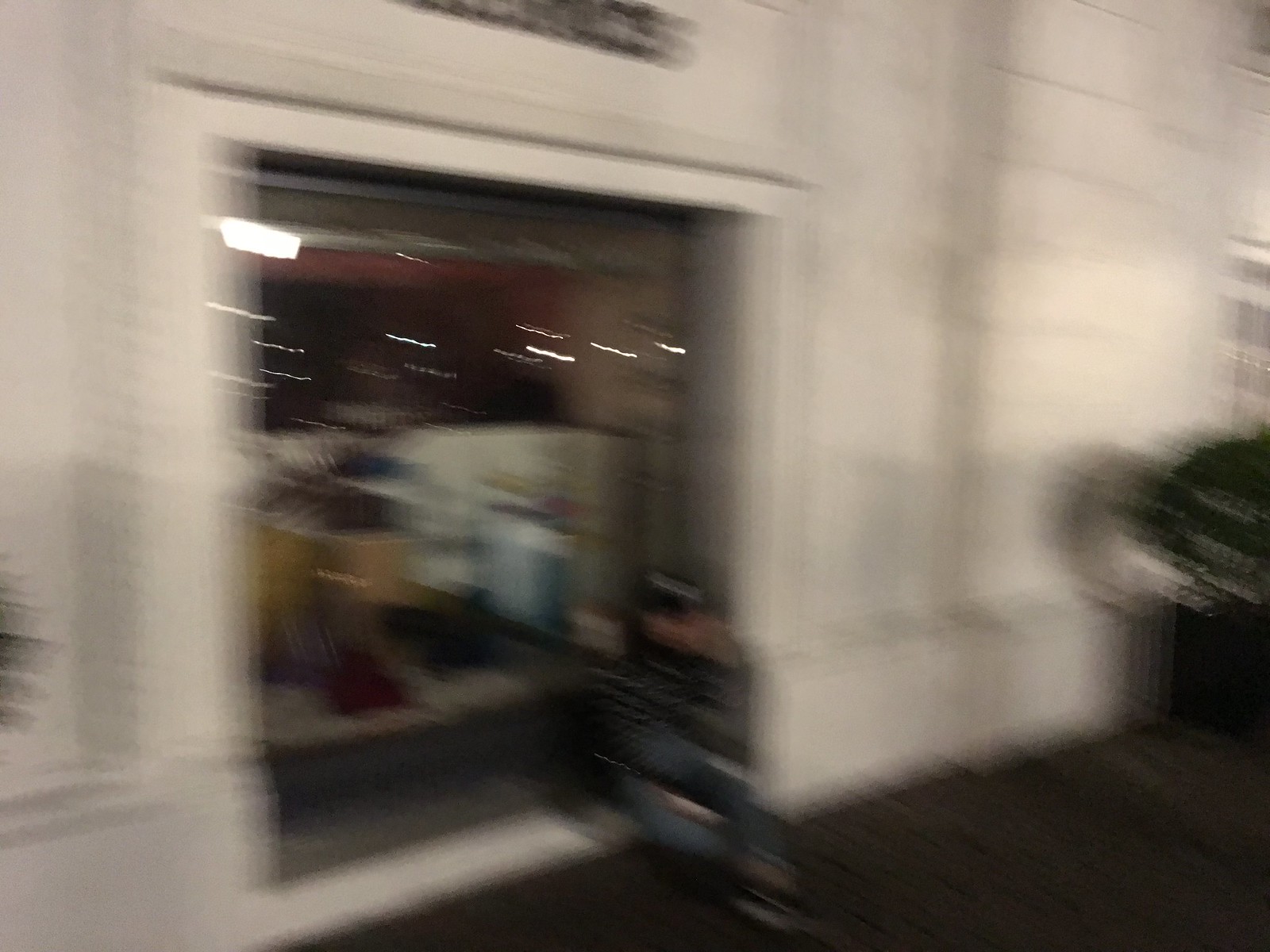The image is a highly blurry color photograph, with an unclear subject matter. It appears to depict a white building featuring a large, glass display window slightly left of center. Inside the display window, there are indistinct shapes that could be mannequins. In front of the window, there seems to be a person seated, though the details are unclear due to the blurriness. The bottom right corner of the image is obscured by a black section, and there is a similarly indistinct black object along the right edge of the photograph. Above the large glass window, there is some illegible writing. Overall, the image lacks fine details and is difficult to decipher due to its poor quality.